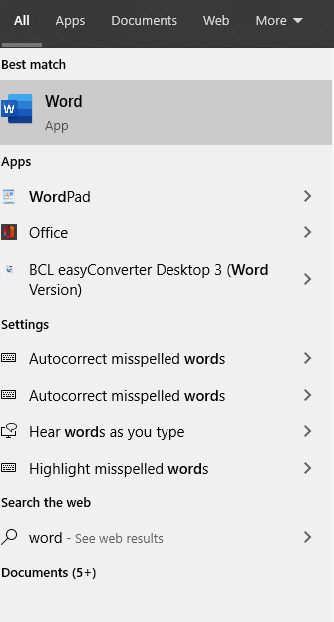This image is a screenshot of a mobile application’s search interface in portrait orientation. At the top, there is a horizontal black bar featuring a white-font title "All," which is underlined in gray. Adjacent to "All," there are additional categories listed in gray font: Apps, Documents, Web, and More, with "More" having a drop-down arrow next to it.

Beneath this bar, the background is white, displaying a list of app suggestions. The first suggestion is Microsoft Word, labeled 'Word,' accompanied by an icon of the Microsoft Word logo to the left, all encased in a gray box. Below this, another section titled 'Apps' includes suggestions such as WordPad, Office, BCL Easy Converter Desktop 3, and Word Version. Each of these app suggestions features an icon to the left and a right arrow, indicating that more information or options are available when clicked.

Further down, there is a 'Settings' section which includes options such as 'Autocorrect misspelled words,' 'Hear words as you type,' and 'Highlight misspelled words.' Each of these settings can be toggled on or off.

At the bottom, there is an option to 'Search the web,' with a search icon and the label 'Word,' inviting users to see web results. Below this, there is a 'Documents' section denoted with the label '5+,' suggesting that more document-related options can be expanded and explored.

Overall, the interface is designed to provide various interactive elements, allowing users to expand and delve deeper into app suggestions, settings, and document-related tasks.